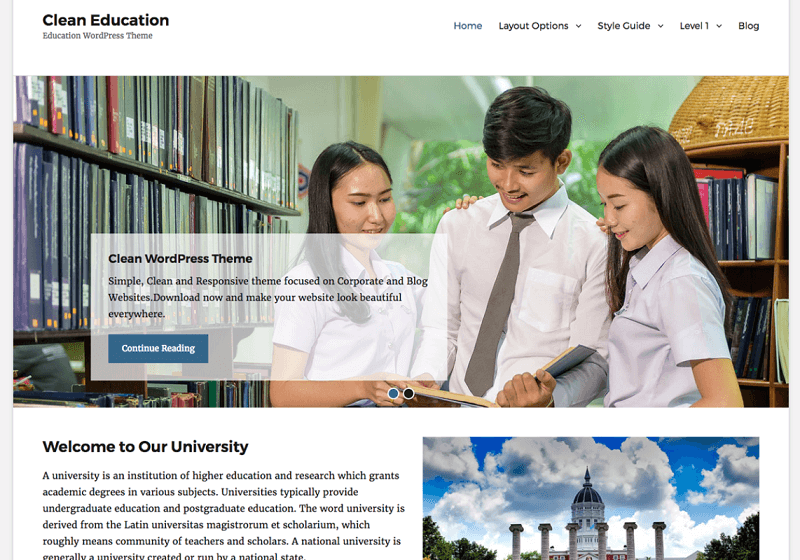This image captures a webpage designed with an emphasis on clean, educational aesthetics. The orientation is landscape, featuring a predominantly white background with a centrally positioned photograph. At the top of the webpage, a horizontal white header spans across the screen. On the left side of this header, in bold black font, the text "Clean Education" is displayed, with "Education WordPress theme" written beneath it in smaller font. To the right side of the header, several navigation links are presented. The word "Home" is highlighted in blue, followed by "Layout options" and "Style guide level one," each with dropdown menus, and finally "Block."

Beneath the header is a landscape photograph set within the white background. The photo appears to be taken in a library, where a bookshelf is visible on the left side. In the center of the photograph, three young children are featured; two girls flank a boy who stands in the middle. The boy is dressed in a white button-down shirt paired with a grey tie, while both girls are wearing white polo shirts.

Below the photograph, another horizontal white bar spans the page. In this bar, a bold black header reads "Welcome to our University," followed by a block of introductory text. To the right of this text is another picture depicting a clear blue sky with large, fluffy white clouds. Dominating the foreground of this image is an imposing building with a tall, dome-like top and a classical facade characterized by six beige pillars. The building's exterior is primarily red brick, lending a stately and scholarly appearance.